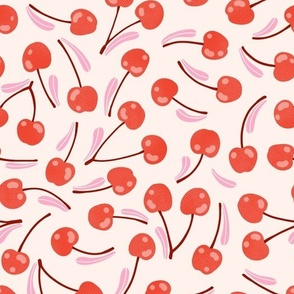The image depicts a decorative design resembling wrapping paper, featuring a repeating pattern of vibrant red maraschino cherries with black stems, set against a background that transitions between light pink and almost white. The cherries are scattered throughout the image in both vertical and horizontal orientations, with some cherries depicted as connected pairs while others float individually. Adding to the whimsical and feminine feel, the design includes deeper pink, feathery, smeared streaks, reminiscent of lipstick or nail polish, which appear randomly across the pattern. Each cherry is carefully illustrated with lighter red highlights to suggest light reflection, and the overall arrangement gives the piece an artistically random yet cohesive look. The absence of text allows the vivid, playful imagery to be the focal point, making it ideal for decorative purposes, especially as wrapping paper likely intended for girls.